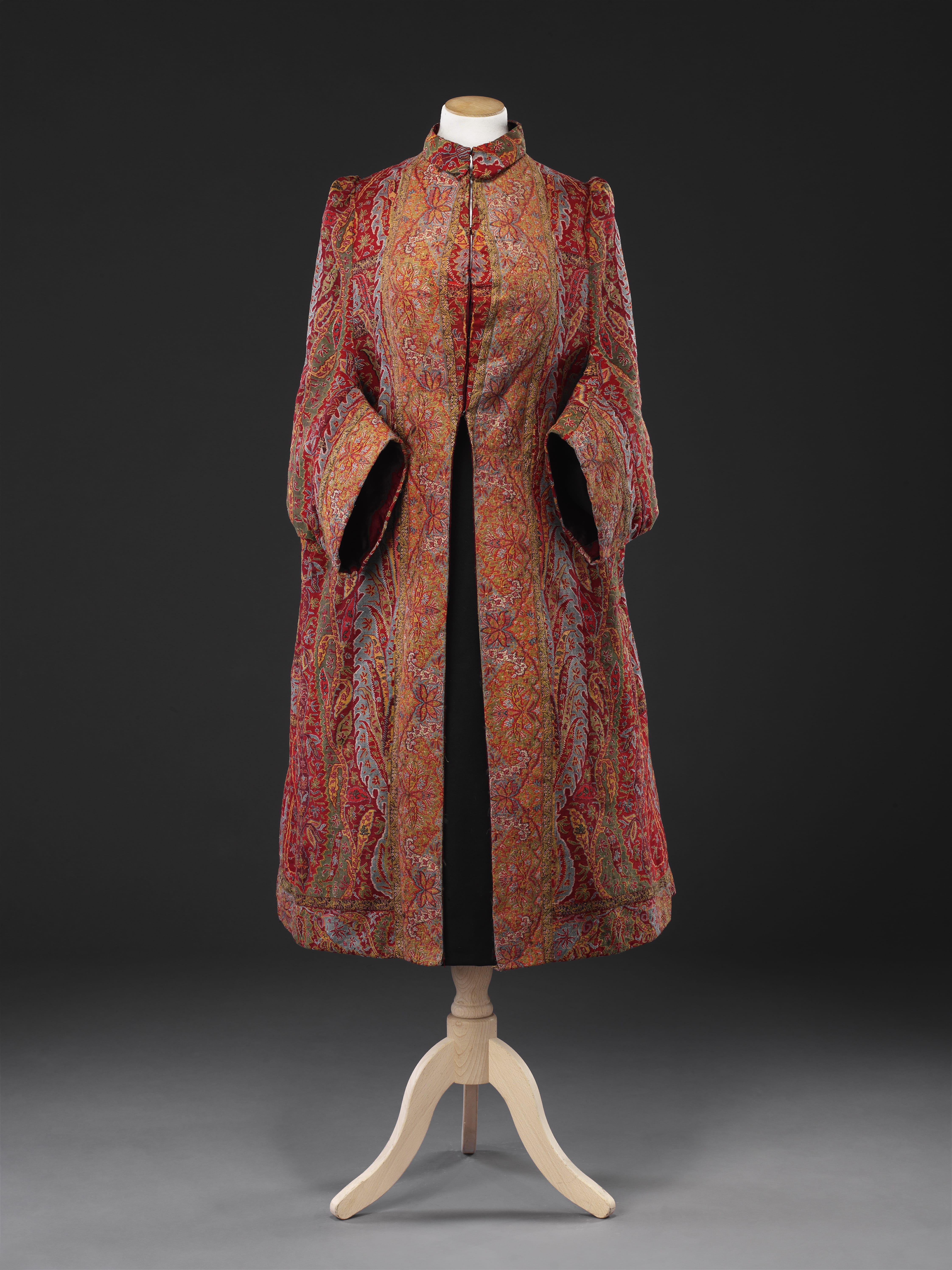This image showcases a traditional, antique-looking, quilted robe with intricate floral and swirl patterns in shades of crimson red, orange, brown, and light blue. The robe, which resembles an Asian-style wizard's coat, hangs elegantly on a headless, white mannequin that is supported by a three-legged wooden base. The base's legs extend outward, stabilizing the display. The robe is ankle-length with loose, wide, and open sleeves. It features frog closures from the chest to the neck, with a slit starting from below the chest extending all the way down. The robe's detailed design incorporates pink flowers with olive and dark green stems, creating a tapestry-like texture. In the background, a diffuse gray setting transitions to near black at the top corners, while the light wooden stand casts a shadow on the gray floor. This piece is displayed in what appears to be a museum, focusing on its historical and artistic significance.